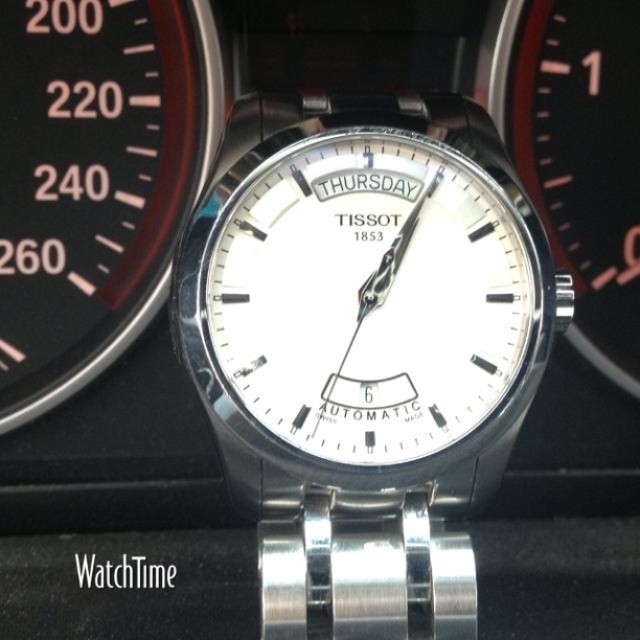A detailed photograph showcases a sleek silver Dysot 1853 watch with a white face, prominently displaying "Thursday" at the top. The watch face reads 1:05, and the second hand is poised at the 34-second mark. The bottom of the dial features the word "automatic" beneath the numeral 6. The scene is set within a vehicle, likely on the driver’s side dashboard, as indicated by the background elements, including a speedometer marked with increments of 200, 220, 240, and 260 (assumed to be in kilometers). The odometer indicates numbers 1 and 0. Both the speedometer and odometer have black faces with chrome borders, against a predominantly charcoal dashboard, highlighted by segments of red metal. The caption “watch time” is subtly placed on the bottom left-hand side of the photograph.